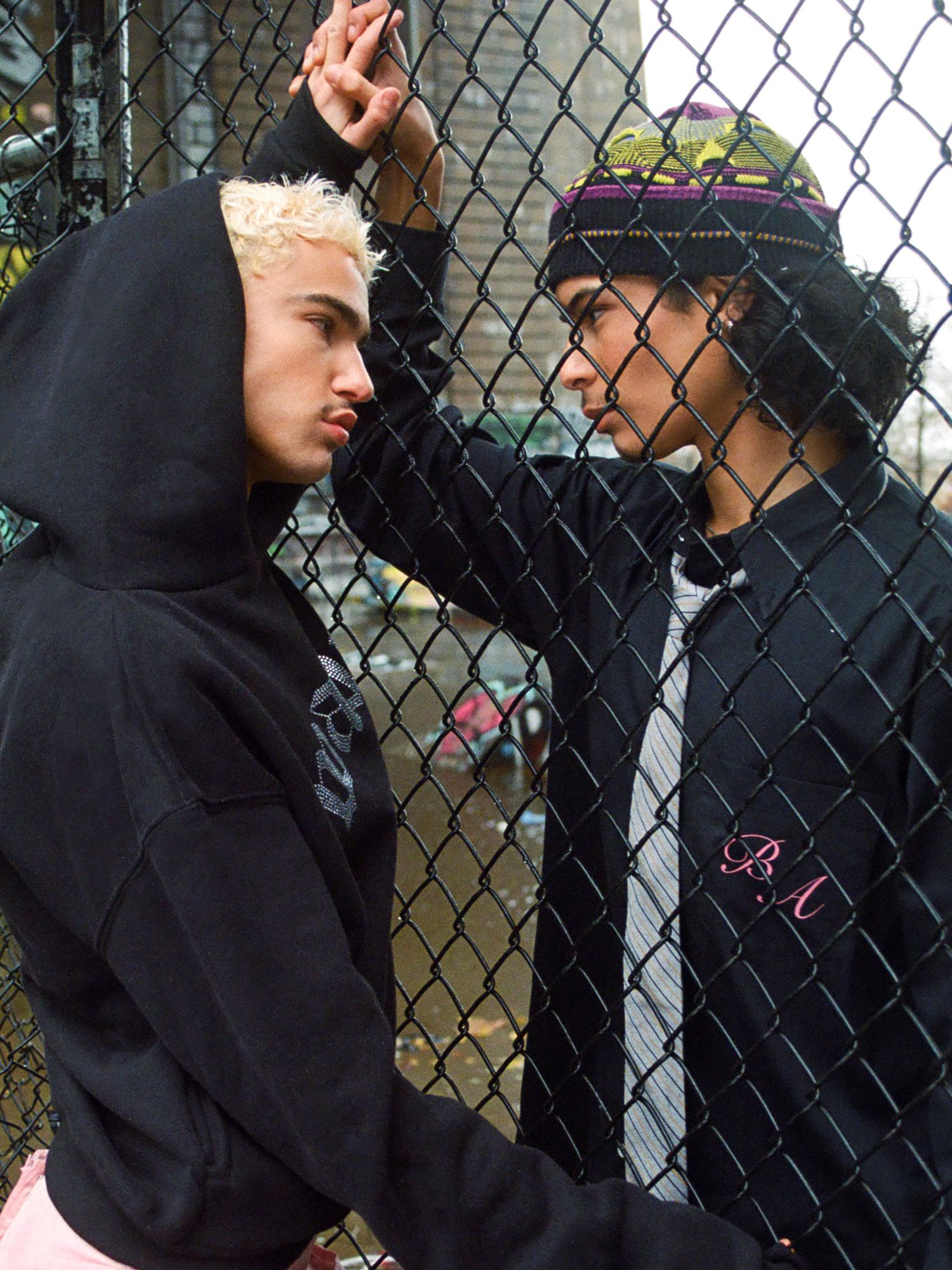This is a vertically rectangular, full-color, staged photograph taken outdoors during the daytime. Two individuals are separated by a black chain link fence, standing waist-up in the frame and gazing directly into each other's eyes. In the background, you can see a grassy area, the wood siding of a large building, and the sky, which appears more white on the upper right side.

On the left is a person who appears male, with bright bleached blonde hair partially covered by a dark black hoodie. This individual has thick black eyebrows, a slight mustache, and a distinctive black mole above his right lip. His left hand is interlinked through the fence with the other person’s hand.

The person on the right has brown skin and brown curly hair, largely concealed by a colorful wool hat featuring a black band with orange dots and a mix of purple, green, and yellow. This individual wears a black jacket adorned with pink initials “B.A.” on the chest, and underneath, they have a grayish-white shirt and a black t-shirt. While holding hands through the fence, they both maintain an intense, direct eye contact.